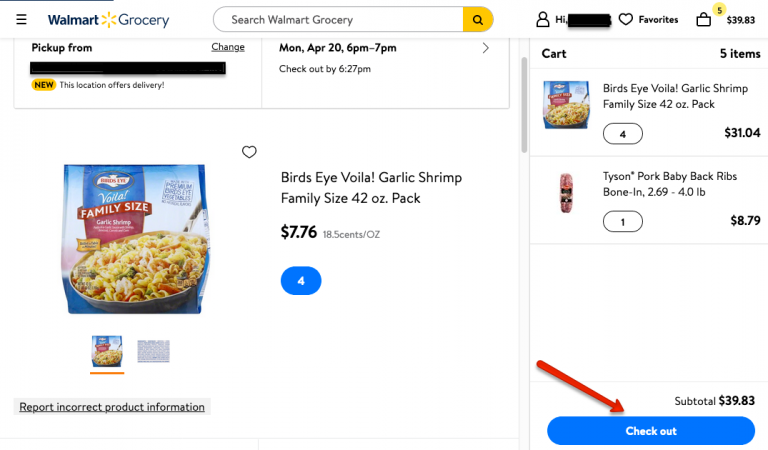Sure, here is a cleaned-up and detailed caption for the image:

---

The image showcases the webpage of Walmart Grocery's online shop. At the top left corner, a blue text reads "Walmart Grocery" with a star icon nestled in the center. The background of the entire webpage is white. On the right side of the page, a cat graphic is situated with the website’s products prominently displayed on the left.

At the top of the webpage, a search box is evident, bearing the prompt "Search Walmart Grocery," and flanked by a yellow search button. To the top right, icons for the user profile and favorites are visible, with the user profile icon obscured in black color. Below these icons, the cat icon indicates there are five items in the cart, displayed in a combination of black text and a yellow circle. The total cost of the items in the cart is prominently shown as $39.83.

On the main page, toward the left side, a specific product is highlighted. The product is "Birds Eye Voila! Garlic Shrimp Family Size" in a 42-ounce pack priced at $7.76, equating to 18.5 cents per ounce. The product quantity is marked as four. Over the product, the text "Pick up from" appears, with the location address concealed. This location offers delivery from Monday, April 20th, between 6 p.m. to 7 p.m. There is also a small insertions indicating the selection of the checkout time slot from 6 p.m. to 7 p.m. The product’s image is positioned on the left side, showcasing the packaging in blue with a visually appealing yellow pan of food.

To the right, the cart section reiterates having five items. A breakdown of the cart contents lists four "Birds Eye Voila! Garlic Shrimp" totaling $31.04 and a "Tyson Pork Baby Back Ribs" priced at $8.79. The subtotal amounts to $39.83. At the bottom right corner, a blue checkout button with white text saying "Check out" is prominent, highlighted further by a red arrow pointing towards it.

---